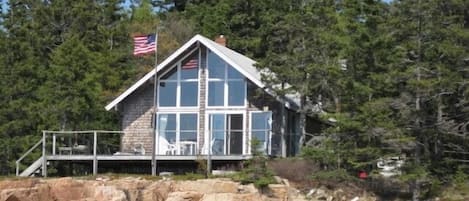This photograph captures the exterior of a modern, detached house situated in a striking, rural location. The house, which features a unique five-sided design with triangular roofs converging at a central point, occupies the center of the image. Dominating the front facade are extensive floor-to-ceiling glass windows on both the ground and first floors, framed in white and accompanied by sliding doors. The lower part of the building is constructed from gray-colored brick, harmonizing with the large gray patio that extends in front of it.

In the forefront of the image, a tall silver flagpole stands on a bed of tan and brown rocks, displaying a fully extended American flag—a sign of a windy day. Adjacent to the flagpole is a cozy seating area on the deck, furnished with a small table and chairs, suggesting a space for outdoor relaxation. The picturesque setting is further enhanced by the presence of towering evergreen trees, notable for their striking green color, that flank the house, framing it against the natural backdrop. In the bottom left corner of the photograph, a white stone cliff subtly enters the frame, emphasizing the house's cliffside position. This isolated, cabin-style home presents a blend of modern architecture and serene, natural surroundings.